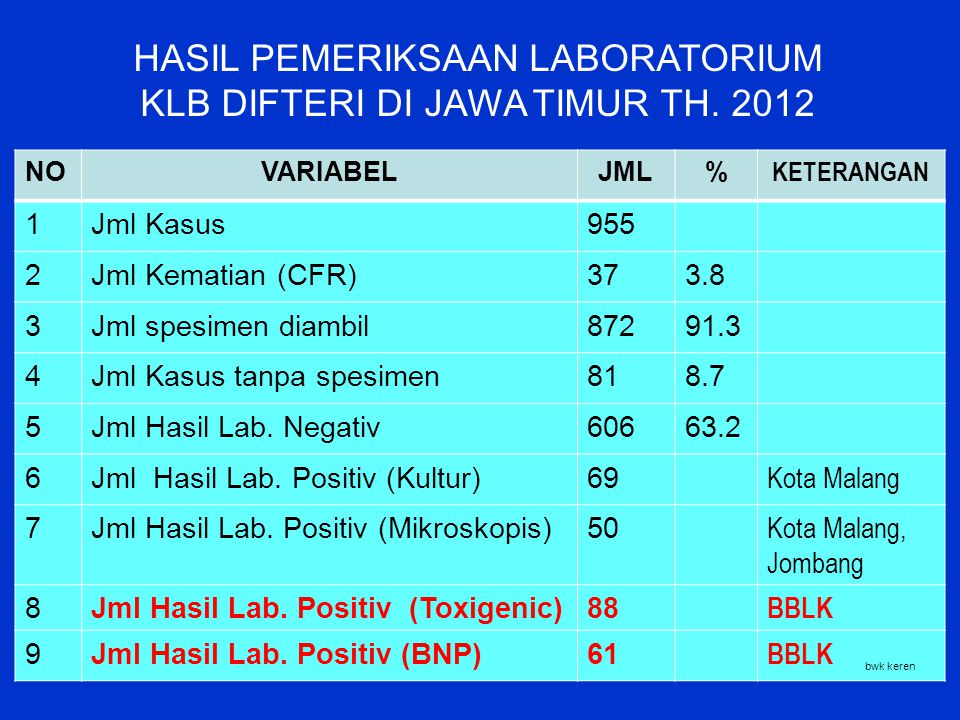The image features a detailed chart from a 2012 presentation on a diphtheria outbreak in East Java, Indonesia. The rectangular chart is bordered by a dark blue outline with a broader top section that houses the chart's title in white uppercase letters: “HASIL PEMERIKSAAN LABORATORIUM KLB DIFTERI DI JAWA TIMUR TH 2012," which translates to "Results of Laboratory Examinations for Diphtheria Outbreak in East Java, 2012." The chart itself has a turquoise and aqua background with black lettering. It consists of nine rows and several columns labeled "Number," "Variable," "JML," "Percentage," and "Keterangan."

Each row, numbered 1 through 9, details different aspects of the outbreak. The columns highlight statistical elements such as the total number of cases (995), number of deaths (37), and various laboratory results. Key data points include:

- 995 total cases.
- 37 deaths (CFR 3.8%).
- 872 specimens taken (91.3%).
- 81 cases without specimens (8.7%).
- 606 negative lab results.
- 69 positive lab results by culture.
- 50 positive lab results by microscope.
- 88 positive toxigenic results.
- 61 positive BNP results.

The chart uses technical terms such as "JML" indicating the number of cases and "Keterangan" for further explanations, which include terms like "Cotamalang" and "BBLK." The detailed breakdown provides a comprehensive snapshot of the outbreak's laboratory findings and case distribution in the region.